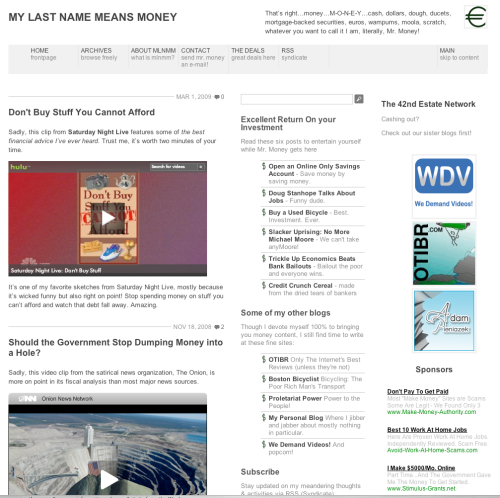**Detailed Caption for the Screenshot of the Website:**

The image depicts a screenshot of a portion of a website with a solid white background, heavily populated with text and various interactive elements. The small, dense text scattered throughout the page makes readability difficult.

In the upper left corner, the text "my last name means money" is prominently displayed in black font. Moving to the right, near the top right corner, there is an extensive block of text about money, though it's not easily legible. The very top right corner features a distinctive icon resembling a circle with two lines through it.

Directly below this section, a horizontal gray navigation bar stretches across the page, offering clickable options labeled "home," "archive," "about," "contact," "deals," "RSS," and "main."

The left column of the screenshot includes multiple sections. First, there is a bold directive, "Don't buy stuff you cannot afford," followed by accompanying text and a clickable video link. Below this, another segment poses the question, "Should the government stop dumping money into a hole?" accompanied by text and another video link.

The middle column includes a text bar for searching, below which is a heading that reads, "Excellent return on your investments." This section is supported by text and various clickable links. Towards the bottom of this column, there's a section titled "some of my other blogs" that includes more text and additional clickable links.

The rightmost column is labeled "The 42nd Estate Network" and contains textual content along with two to three small clickable images for sponsors. The bottom right of this column houses at least three sponsored links, providing further navigation options.

Overall, the screenshot captures a highly detailed and intricate webpage, designed with numerous sections, clickable elements, and a predominant theme centered around financial advice and investments.